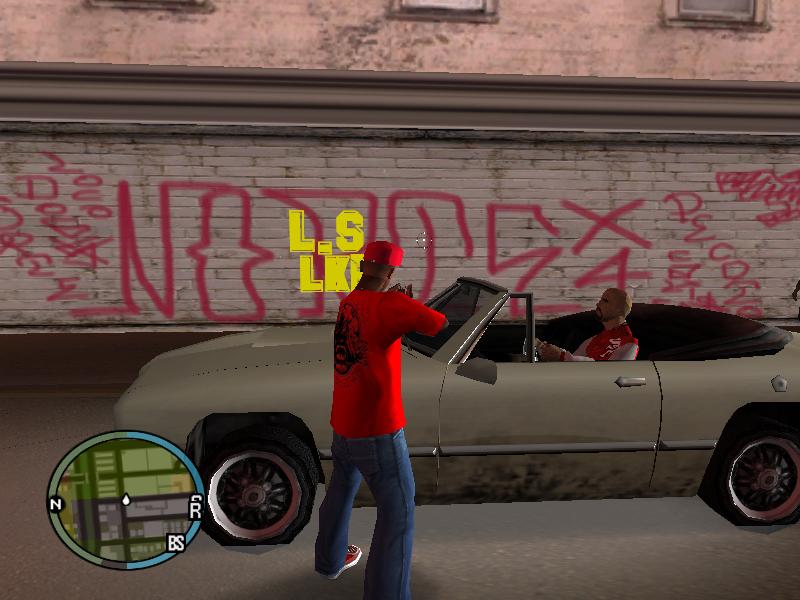Screenshot from a video game reminiscent of Grand Theft Auto, featuring a player character named LSLKE. The character, who appears to be African American, is dressed in jeans, red sneakers, a red t-shirt, and a red ball cap. He is seen aiming a gun at a passing convertible with a male driver. In the background, a gray brick wall is prominently covered in various graffiti, adding to the urban atmosphere of the scene.